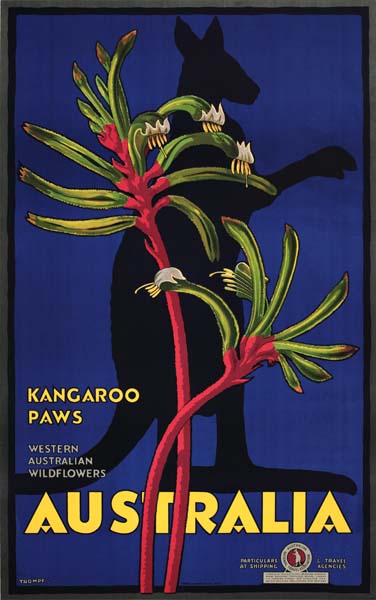This poster is a tall rectangular image with a thick dark gray border and an inner thick black border. The background features a deep blue color, resembling a painting. Dominating the bottom of the poster, the word "Australia" is boldly displayed in yellow letters with black borders. Above this, a giant black silhouette of a kangaroo stands on its hind legs, facing right with its arms extended towards the top right corner, and its tail extending left out of the image. Overlapping the kangaroo is a striking painting of a wild plant, known as "Kangaroo Paws," showcasing a tall red stalk and another bent stalk with green spikes at the ends. The poster also advertises "Western Australian Wildflowers," emphasizing the unique flora of the region. In the bottom right corner, there appears to be an emblem featuring a kangaroo with some text, further promoting the wild wonders of Australia.